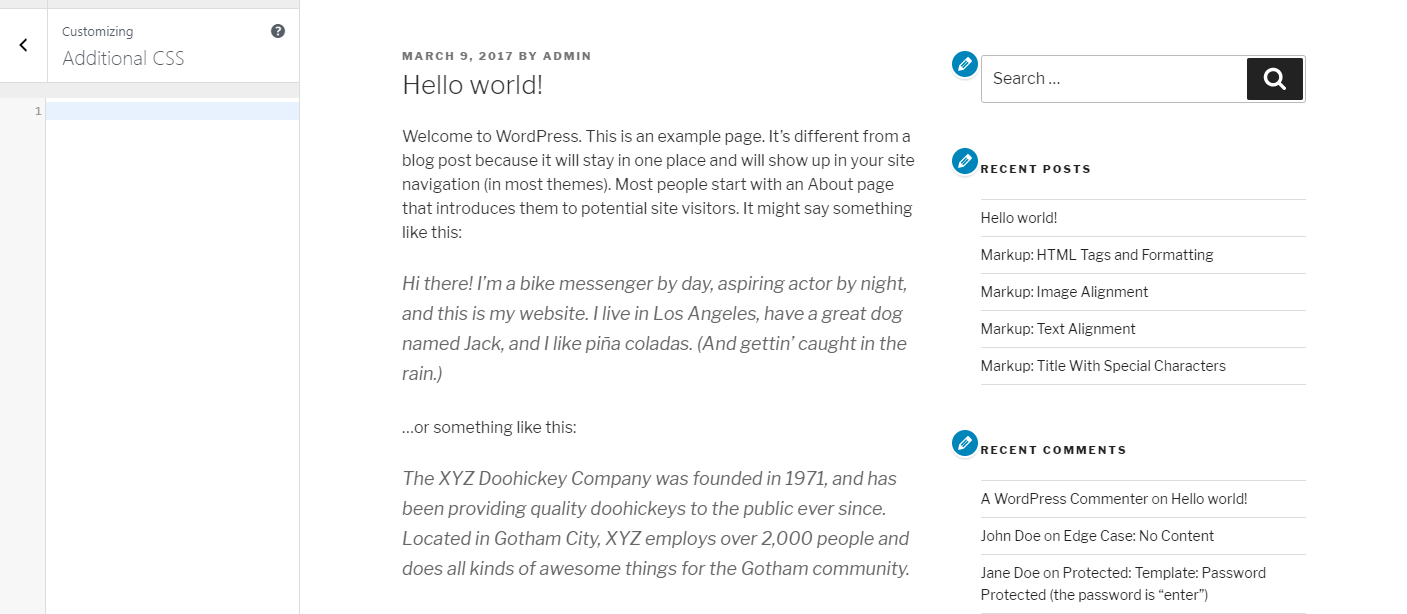The image depicts the upper left section of a webpage where additional CSS customization options are available. A question mark inside a black circle indicates help or guidance, dated March 9, 2017, with a post by the admin titled "Hello World." The content is part of a WordPress site, showcasing an example page that remains static unlike blog posts, and is typically included in site navigation.

The introductory text on the site presents two examples of what an "About" page might contain. The first example introduces a fictional character, a bike messenger by day and an aspiring actor by night, living in Los Angeles with a dog named Jack. It humorously adds the character's interests in pina coladas and getting caught in the rain. 

The second example describes the XYZ Doohickey Company, established in 1971, known for producing high-quality doohickeys. The company is located in Gotham City, employs over 2,000 people, and contributes positively to the local community.

On the right side of the image, a search bar is displayed, along with sections for recent posts, recent comments, and entries for HTML tag formatting, image alignment, text alignment, and titles with special characters. Each entry in these sections is accompanied by a blue circle with a pencil icon, indicating that they can be edited.